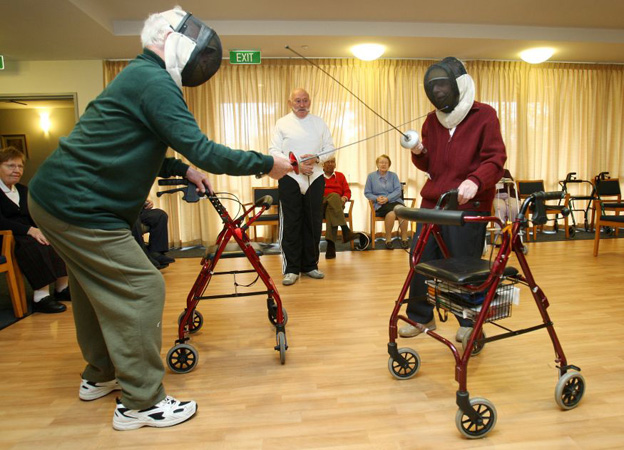This vivid color photograph captures an intriguing indoor scene of two individuals engaged in a unique form of fencing. The setting, which resembles a nursing home or a facility for individuals with disabilities, features a wooden floor, yellow ceiling lights, and yellow-draped windows. 

At the center of the image, two participants are poised for action. The person on the left is dressed in a green top with lighter green trousers and trainers, while the person on the right sports a red top with matching reddish trousers. Both individuals, who appear to have dark skin, are wearing protective helmets with white padding on the sides and back. They each hold a red walker or rollator in their left hand, and their swords are crossed, suggesting an imminent fencing duel. 

In the background, additional rollators are visible, emphasizing the setting’s support for mobility. A row of chairs lines the back of the room, with a couple of people seated and observing the activity. A bald man, dressed in a white top and shorts over black trousers and possessing lighter skin, stands between the participants, possibly facilitating or refereeing the match.

An exit sign is prominently displayed behind the group, providing a point of reference within the room. To the right, another man with lighter skin watches the scene unfold, adding to the atmosphere of curiosity and engagement.